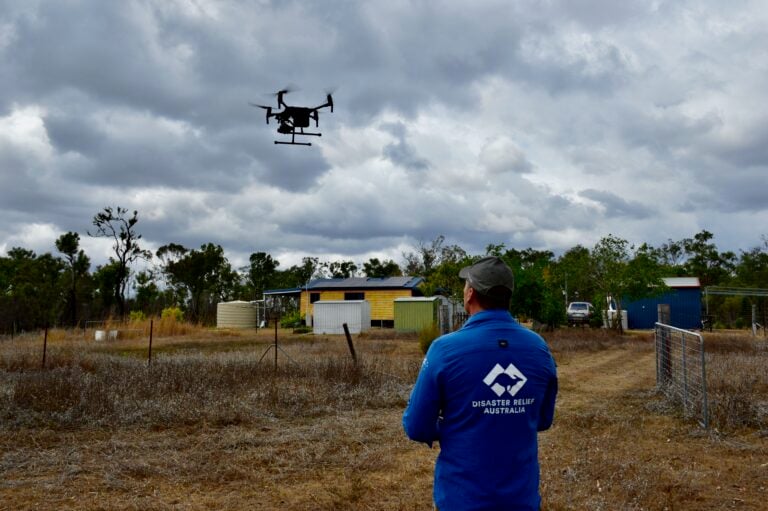In the image, a man is seen operating a drone, positioned towards the lower right with his back facing the camera. He is wearing a blue jacket with the text "Disaster Relief Australia" in white, and a logo featuring an overlapping diamond pattern with an outlined kangaroo. The man also has on a dark grey baseball cap. The scene is set in a farm-like environment with tall, dry, brown grass and dirt. Surrounding him are various structures, including a small yellow house with wood paneling, sheds, and outbuildings, all bordered by a chicken wire fence and additional fencing to the right. In the background, a line of trees under a cloudy, grey sky completes the pastoral landscape. The black drone hovers around 20-30 feet above the ground, featuring four propellers and landing rods for stability. The man appears to be looking up at the drone he is controlling, amidst this distinctly Australian setting characterized by sparse vegetation and rural elements.